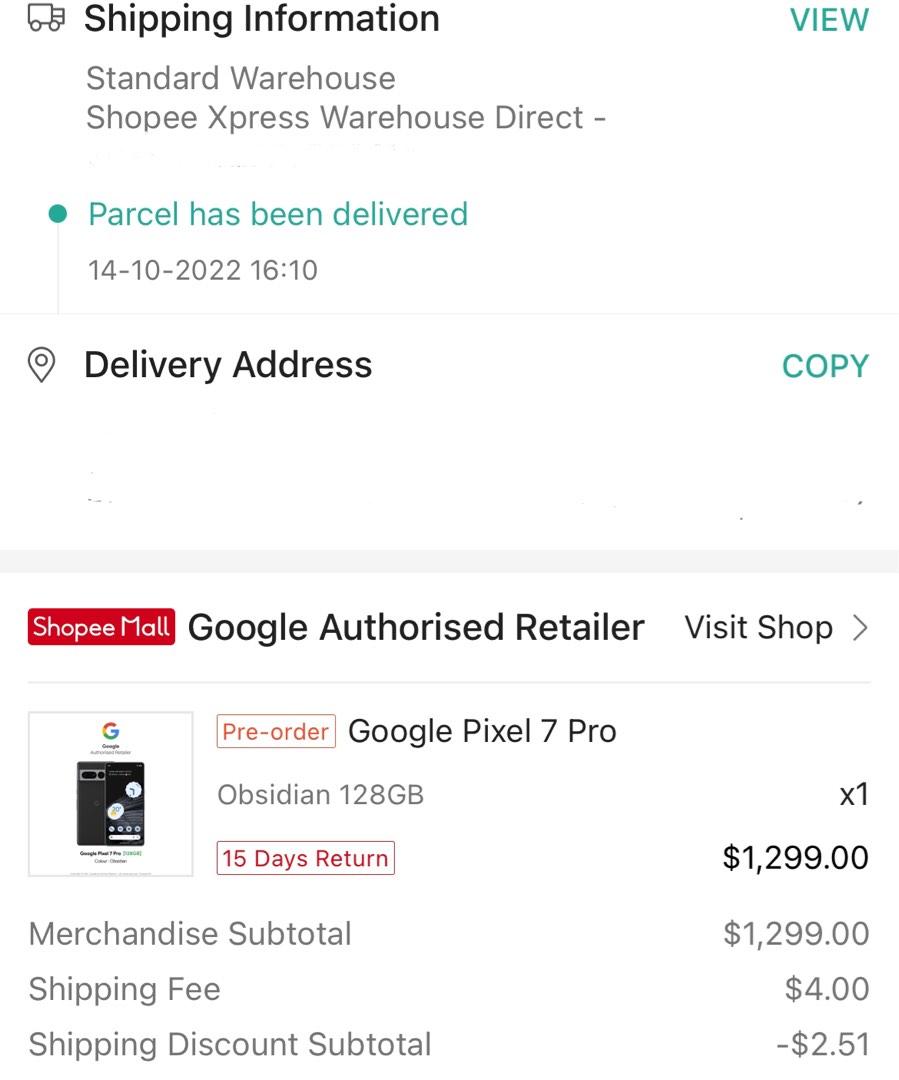The image depicts a detailed summary of an order page.

At the top half of the page, a light gray horizontal border, approximately a quarter of an inch thick, separates the white background above and below. In the top left corner, there is an icon of a shipping truck, followed by a bold black label that reads "Shipping Information." Adjacent to this, on the right side, a label in blue capital letters says "VIEW." Below the "Shipping Information" label, a slightly lighter black text denotes "Standard Warehouse," followed by a line that reads "Shop EE Express Warehouse."

A small teal dot appears next, accompanied by the text "Parcel has been delivered" to its right. Underneath, in black text, the date and time "14-10-2022 16:10" are specified. Further down, a black-outlined location icon is positioned on the left, with a bold black label "Delivery Address" beside it, and to the right, in teal, the word "COPY."

Below the gray divider line in the middle of the page, a red rectangle on the left displays "Shop EE Mall" in white text. Next to it, the black text reads "Google Authorized Retailer," followed by "Visit Shop" and a greater-than sign (">") pointing right, aligned with a thin gray vertical bar.

Below this, there is a small white square on the left containing a phone image with the Google "G" logo above it. To the right of this square, product information such as storage capacity (gigabytes) and return policy details are listed. On the right side, the cost of the item is displayed.

Underneath this section on the left, details regarding financial breakdowns are detailed in black text, including "Merchandise Subtotal," "Shipping Fee," and "Shipping Discount Subtotal." Corresponding numerical values for each cost element are listed on the right side.

Overall, this page seems to be an organized summary pertaining to a recent order, showcasing shipping details, the product purchased, and the cost breakdown.